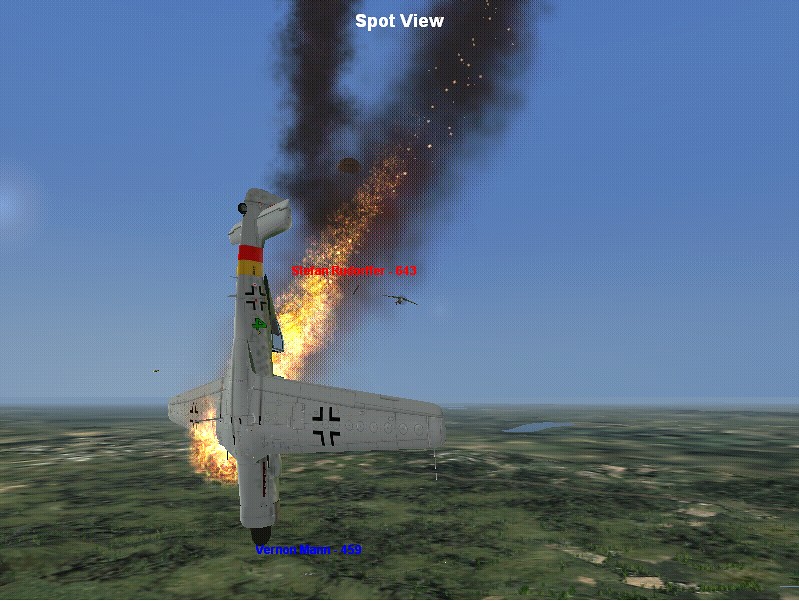The image captures a highly realistic screenshot, possibly from a video game. The upper two-thirds of the frame are dominated by a cloudless, vivid blue sky, accentuating the high altitude of the scene. Below, a patchwork of green lawns, tree canopies, farmland, and grayish rooftops spread out across the landscape, offering a serene contrast to the upper section. At the center of this dramatic image, an airplane is depicted in a perilous nosedive. The aircraft, painted gray with a distinctive red and yellow stripe at the tail, is engulfed in bright orange and yellow flames emanating from one of its wings. Dark smoke trails behind, underscoring the plane’s dire situation. At the very top of the screenshot, a caption reads "Spot View," likely indicating the perspective mode within the game. The scene is both visually striking and evocative, blending serene and chaotic elements seamlessly.